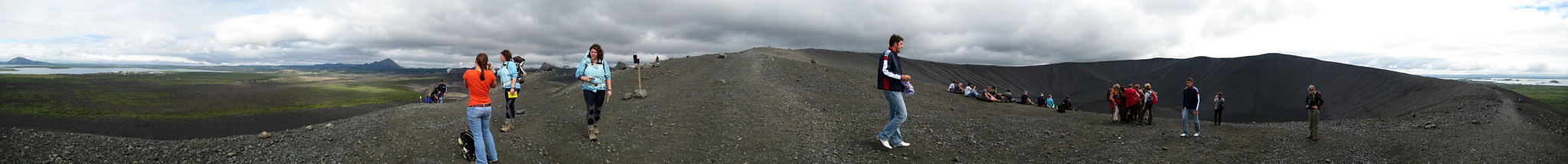The photo, taken outdoors, showcases a panoramic view of a hill or mountaintop predominantly composed of sandy ground. On the right side of this elevation, there's a sizable crater where a significant number of people have gathered, either standing or seated in groups. Another cluster of individuals is seen along the left edge of the hill, standing and possibly gazing at the breathtaking scenery. At the center of the image, a man dressed in blue jeans, white shoes, and a dark blue jacket with red stripes and blue sleeves can be observed walking towards the right. The scene extends into the distance, revealing patches of grassland beneath the hill both on the left and further out, suggesting a transition from the rugged hilltop to gentler grasslands below. Overhead, dark or gray clouds loom, suggesting an impending storm, while the overall high-altitude setting is indicated by low, fluffy clouds. The photo, notable for its thin, stretched panoramic format, offers a glimpse into the serene yet dynamic interactions among people amidst a dramatic landscape.